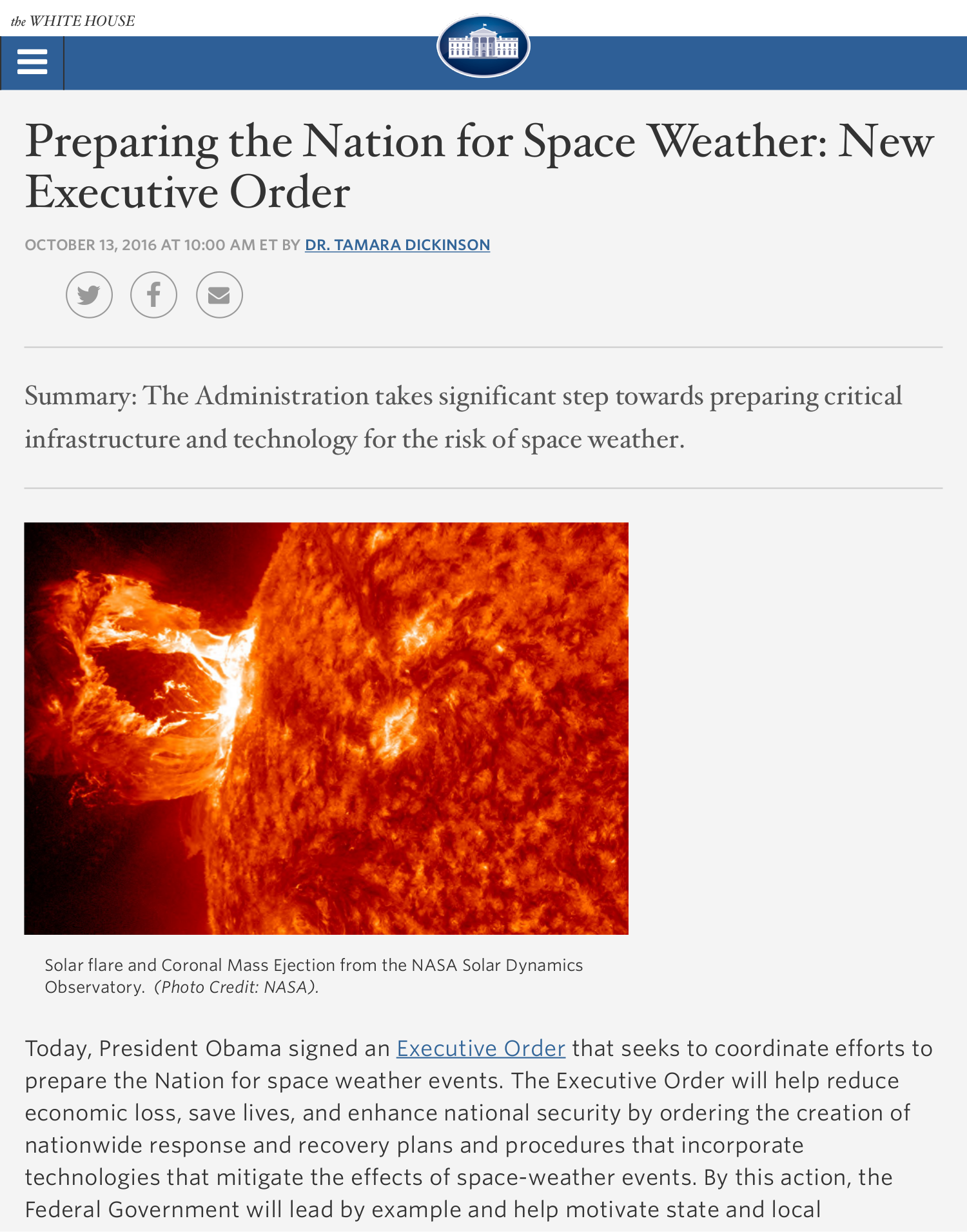This detailed caption accompanies an image of a news article from the White House, adorned with the official White House emblem. The article, titled "Preparing the Nation for Space Weather: New Executive Order," was authored by Dr. Tamara Dickinson and published on October 13, 2016, at 10 a.m. Eastern Time. The piece highlights the administration's significant efforts to ready critical infrastructure and technology against the risks posed by space weather. Accompanying the text is a vivid image of the sun's surface, showcasing a solar flare and a coronal mass ejection, captured by NASA’s Solar Dynamics Observatory. The photo is credited to NASA. The article begins by announcing that President Obama has signed an executive order aimed at coordinating national preparations for space weather events.